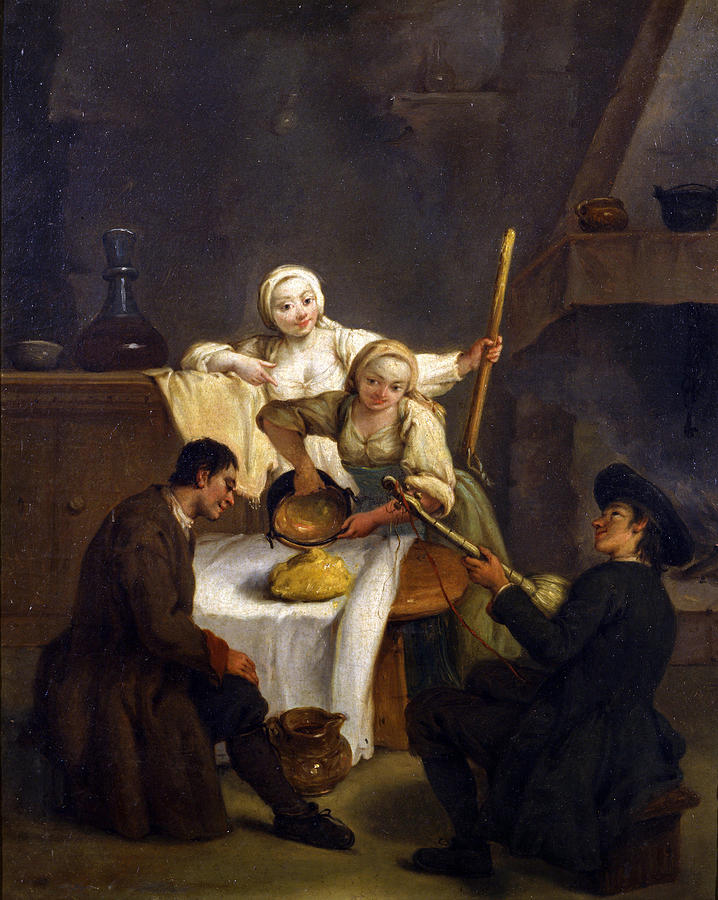This detailed painting likely from the 1800s depicts a dimly lit interior room with rich, dark hues of gray, blue, and brown. Four young adults, appearing to be between the ages of 20 and 25, populate the scene. In the foreground, two men occupy the right side. The man to the right, dressed in all black with a hat, has his back to the viewer and is slightly turning his head leftward and upward while playing a broom-shaped guitar. He stands beside another man with short brown hair, wearing a long brown coat and black pants, who gazes slightly downward. At the feet of this brown-coated man is a pitcher, and next to him stands a wooden table draped in a white cloth. One of the women, facing the camera, stands at this table, pouring some kind of food. She has short blonde hair and wears a white top with a blue apron over a green skirt or dress. In the background, another woman, clad entirely in white with a headwrap and long sleeves, rests her right arm on a dresser, holding a piece of wood in her left hand. The scene suggests a day in the life of kitchen maids and servants, captured with intricate detail and historical authenticity.